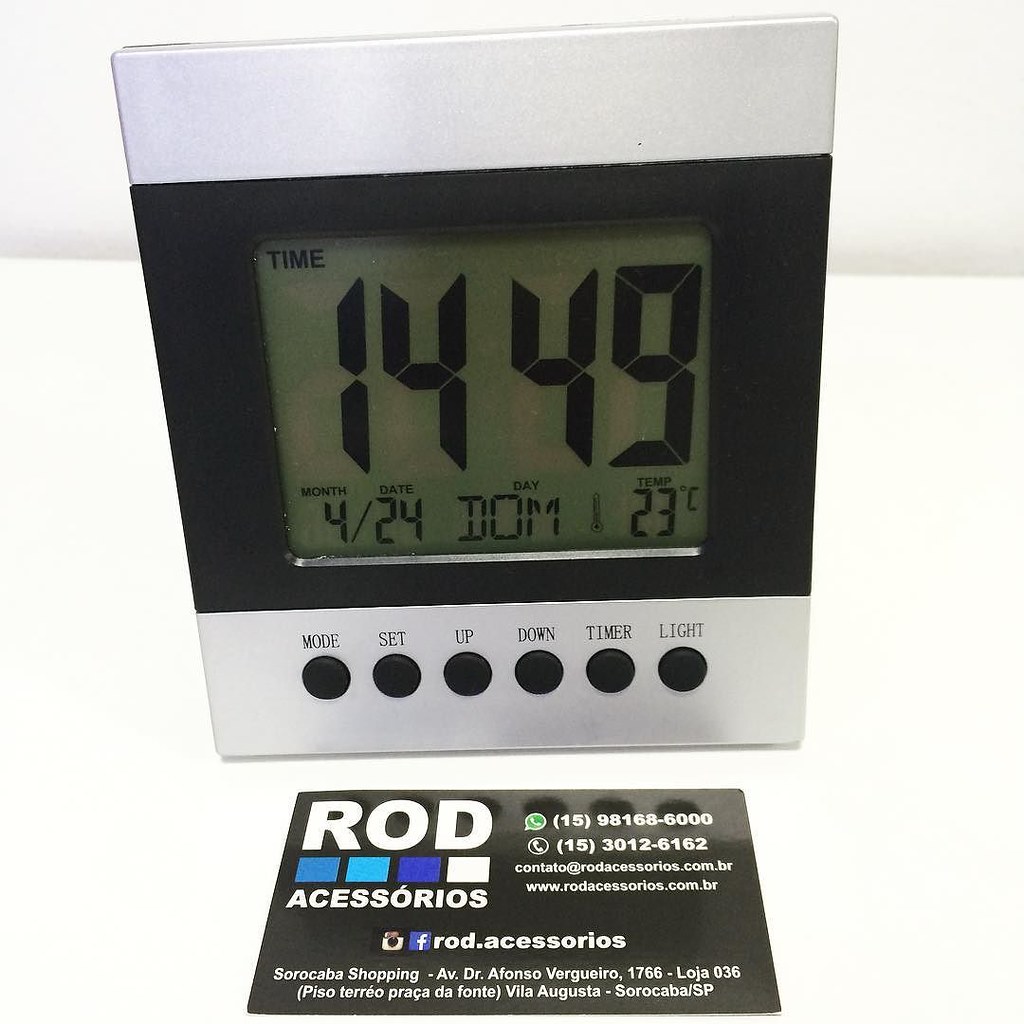The image features a digital clock prominently centered with a sleek, modern design, likely from the mid-2000s. The clock displays the time 14:49 (2:49 PM in non-military time), the date as 4/24, and the day abbreviated as "DOM." The temperature reads 23 degrees Celsius. The clock has a black central display flanked by metallic strips at the top and bottom. Six black buttons labeled "mode," "set," "up," "down," "timer," and "light" are positioned along the bottom metallic strip.

In front of the clock is a business card with a black background. The card features the word "Broad" in white text on the top left, underneath which are four colored rectangles in light blue, dark blue, and white. Below these, it reads "A-C-E-S-S-O-R-I-O-S." The top right of the card lists the phone numbers (15) 98168-6000 and (15) 301-126. The card hints at connections to electronics or accessories, possibly indicated by an Instagram and Facebook logo. The entire scene is set against a plain white background, emphasizing the objects in the foreground.